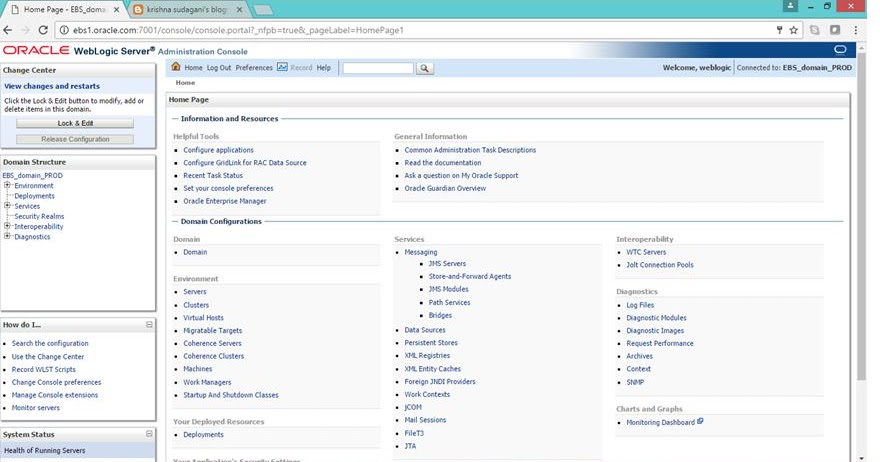**Descriptive Caption:**

This detailed image showcases the user interface of EBS Krishna Sugandani's blog hosted on Oracle WebLogic Server Administration Console, accessible via the URL "EBS1.oracle.com:7001/console/console.portal?_nfpb=true&_pageLabel=HomePage1". 

At the top of the console portal, the tabs reveal two open sections: 
1. The Oracle WebLogic Server Administration Console homepage titled "Oracle WebLogic Server Administration Console."
2. An EBS domain interface where changes can be viewed and restarted through the "Change Center," which allows users to lock and edit for modifying, adding, or deleting domain items.

The left sidebar includes essential tools under the "Domain Structure," grouped as follows:
- Deployments
- Services
- Security realms
- Interoperability
- Diagnostics

There's a functional section offering guidance on "How do I?" to help users with tasks such as searching for configurations, recording WLST scripts, changing console preferences, managing console extensions, and monitoring services.

In the central workspace, the homepage is designed with icons and textual elements, allowing quick access to various features:
- Home, Logout, Preferences, Record, and Help buttons
- A search bar
- Sections for Information Resources, Helpful Tools, Configuring Applications, Grid Link for RAC Data Source, Recent Task Status, and Oracle Enterprise Management

Moreover, there's an in-depth directory under "Domain Configurations" listing:
- Domain Environment components like Servers, Clusters, Virtual Hosts, Migratable Targets, Coherence Servers, Coherence Clusters, Machines, Work Managers, and Startup and Shutdown Classes
- Deployed Resources or Deployments details

At the top, a "Common Administration Tasks" section offers descriptions, documentation references, and support links like "Ask a Question on My Oracle Support" and "Oracle Guardian Review."

Additionally, there are various services detailed, such as:
- Messaging, JMS Servers, Store and Forward Agents, Path Services, Bridges
- Data Sources, Persistent Stores, XML Registries, XML Entity Caches, Foreign JNDI Providers, Work Context, JCOM, Mail Sessions, File, T3, and GTA
- Interoperability tools like WTC Servers and Jolt Connection Pools
- Diagnostics resources including Log Files, Diagnostic Modules, Diagnostic Images, Request Performance, Archives, and Content

Charts and graphs are also available for monitoring purposes on the right side, enhancing the system's visual oversight capabilities.